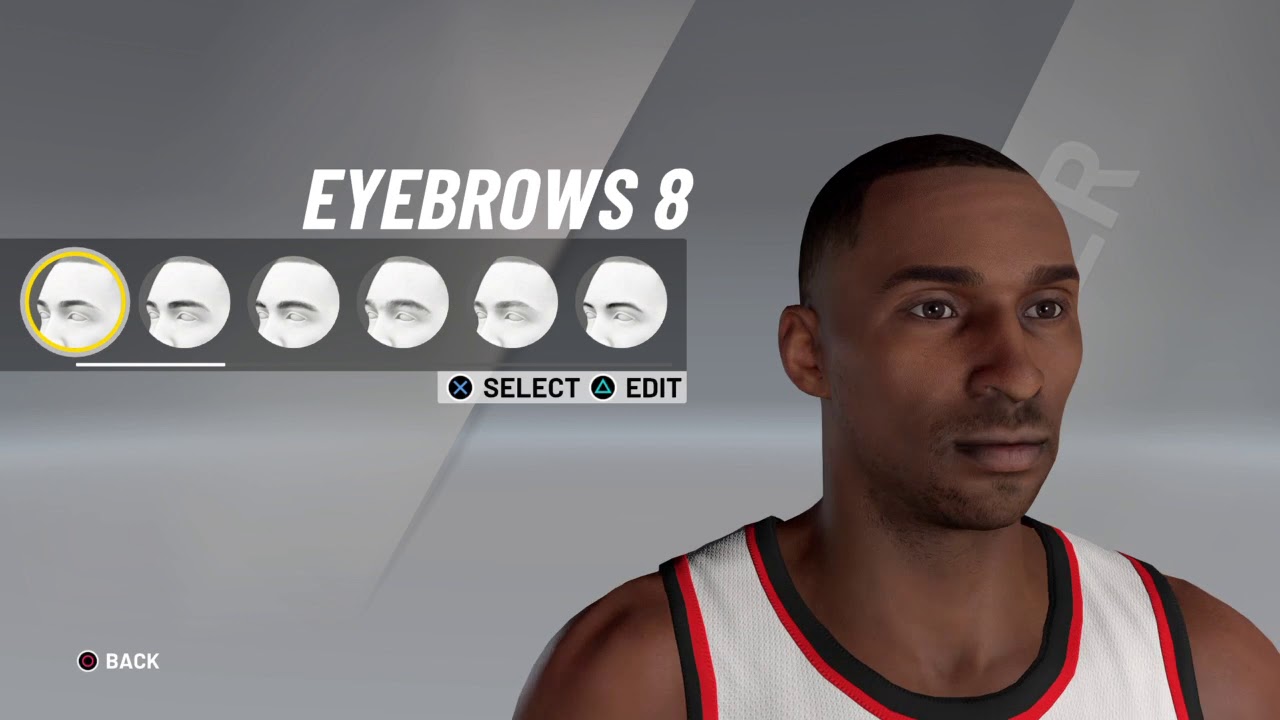This computer-generated image depicts a portion of a web page designed with a gray rectangular background. At the forefront is a professional basketball player, who appears to be African American and likely in his late 20s to early 30s. He is dressed in a white basketball jersey featuring black and red borders. The player sports a short, faded haircut and has light facial hair, including a 5 o'clock shadow, a mustache, and a soul patch.

Text in white, prominently displayed, reads "Eyebrows 8." Below this text are circular images, numbered 1 through 6, showcasing various male foreheads, eyes, and eyebrow styles. Users can select and edit these styles through available tabs. Additionally, a back tab is situated in the bottom left corner, allowing users to navigate back to the previous screen. The purpose of "Eyebrows 8" remains unclear, but it appears to offer customization options for eyebrows.